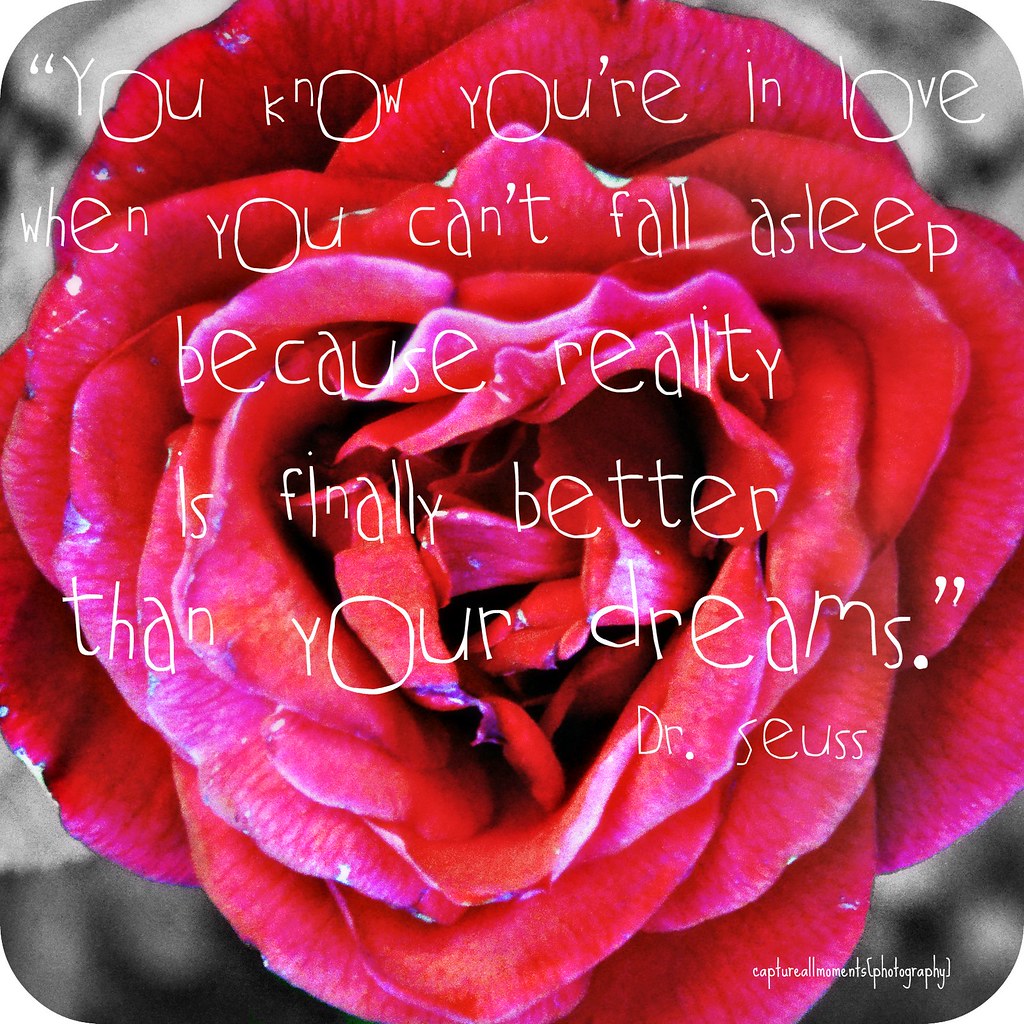The image features a close-up of a rose with a blend of red and pink hues, filling the entire frame. The central focus is on the intricate petals, with an out-of-focus border showing hints of grays and blacks. Overlaying this vibrant background is an inspirational quote in white text: "You know you're in love when you can't fall asleep because reality is finally better than your dreams," attributed to Dr. Seuss. At the bottom right corner, in a distinct font where the vowels, especially the O's, appear unusually large yet not capitalized, reads "Capture All Moments Photography." The combination of the intimate floral detail and the meaningful quote gives the image a poignant and romantic feel.